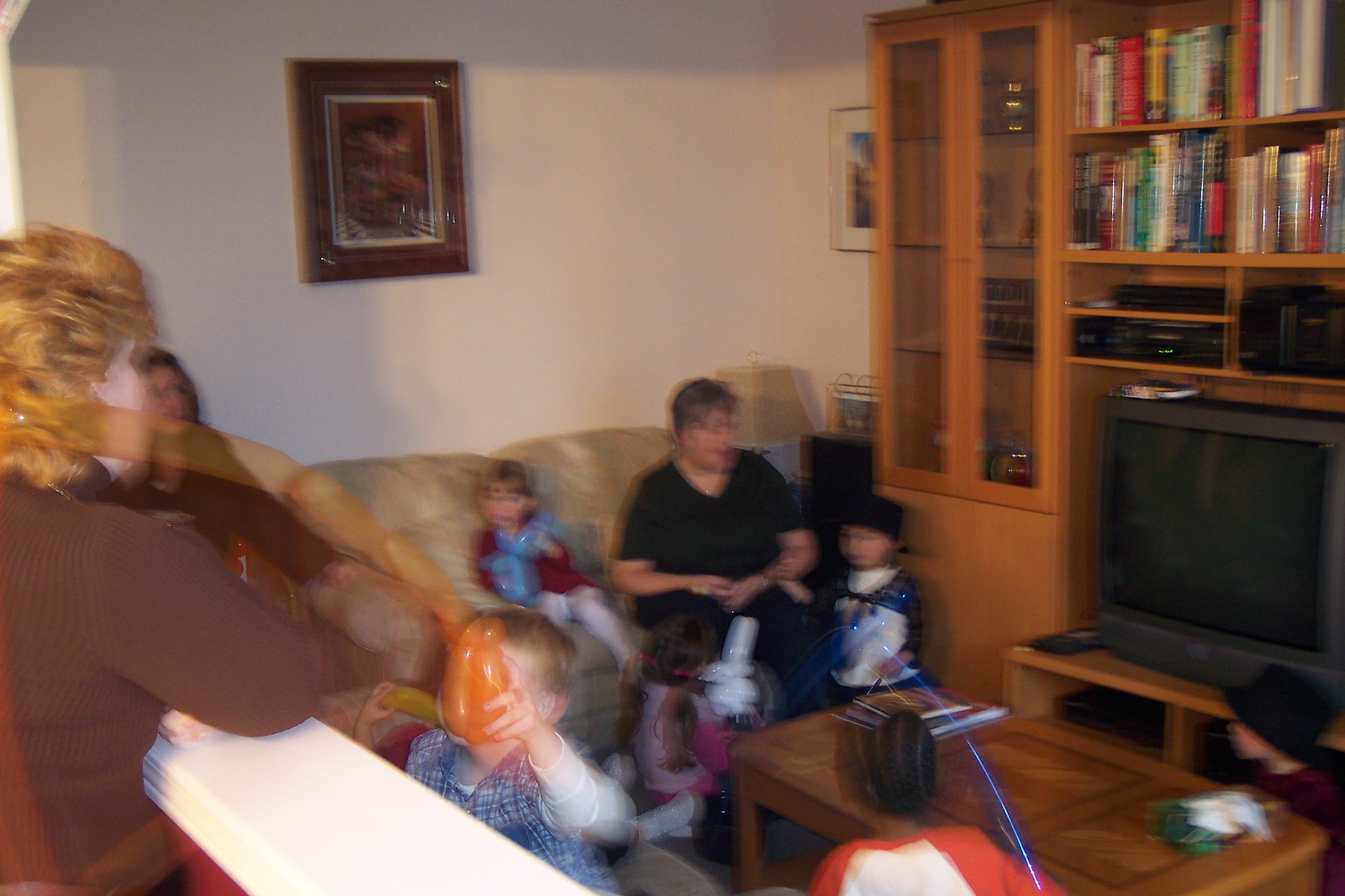This photograph captures a cozy family gathering in a warmly lit living room, though it is somewhat blurred. Dominating the center of the image is a tan-colored couch positioned against the wall. Seated on the couch is a woman with short brown hair, donned in a short-sleeved black t-shirt. To her left is a young girl dressed in a charming red dress with white tights, holding a light blue balloon animal.

To the left of the couch stands a woman with long brown hair, wearing a long-sleeved dark red shirt. Moving closer to the foreground, there is another woman with short blonde hair, dressed in a long-sleeved brown turtleneck. Just beside her, a child with short blonde hair clutches an orange balloon animal. Next to this child, another youngster sports a white and red shirt while holding a dark blue balloon animal.

In the background, a blue-brown coffee table situates itself in front of a large black TV that is part of an entertainment system. An array of books is neatly arranged on shelves above the TV, adding to the homely and lived-in ambiance of the room.